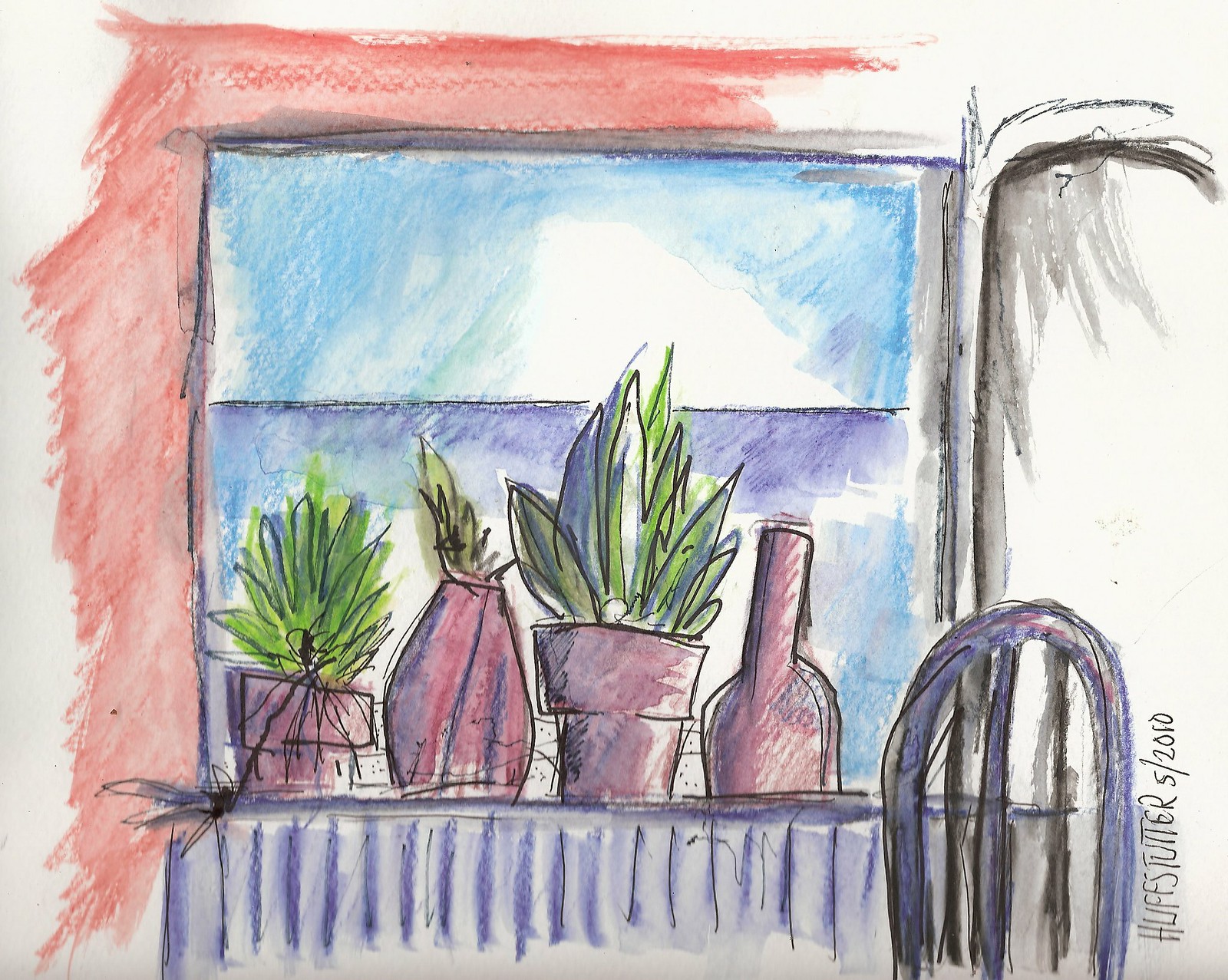This vibrant illustration, executed with colored pens, features a detailed depiction of a windowsill adorned with various plants. The window itself transitions from a blue hue at the top to a purple shade at the bottom, accentuated by a pinkish-orange border. On the purple shelf beneath the window, from left to right, sits a small potted plant with lush green leaves, a bottle with green foliage emerging from it, another potted plant, and a long-necked bottle void of any plant. To the right side of the image, part of a purple chair is visible, adding depth to the scene. The artwork is signed "Huff Setters 5/2010."